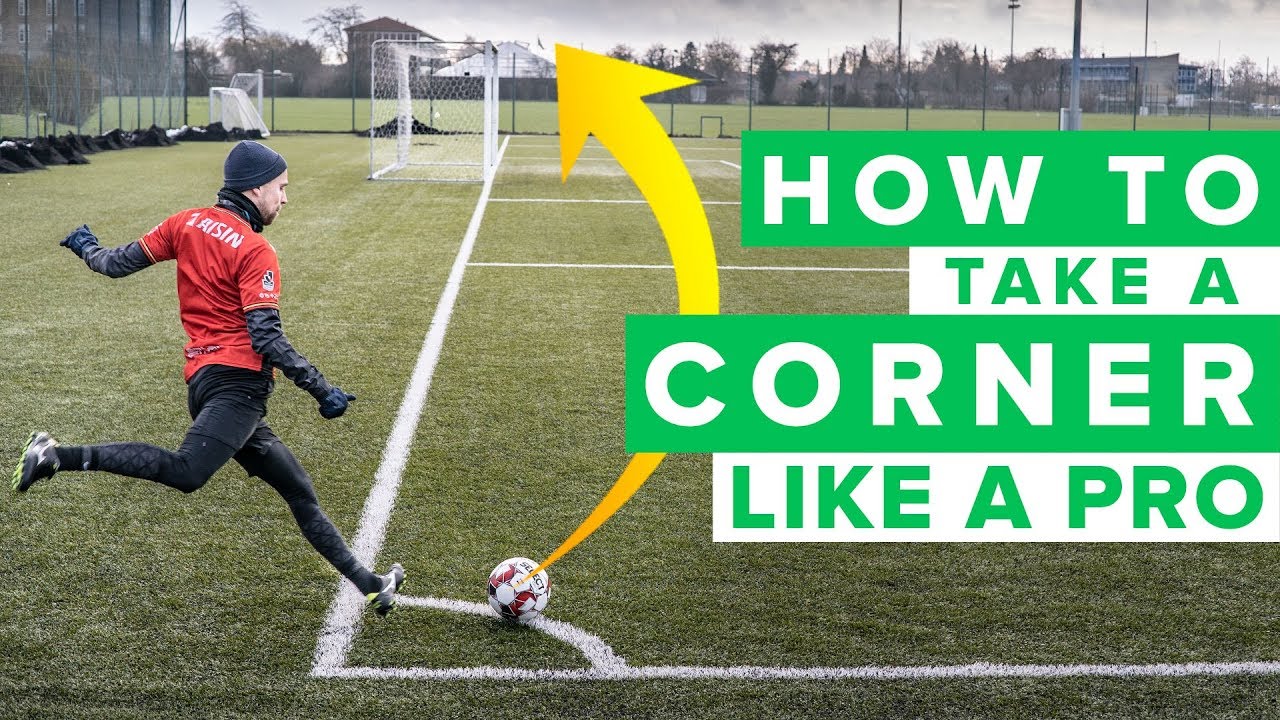The image depicts a soccer lesson titled "How to Take a Corner Like a Pro." Set on an outdoor soccer field, it's positioned at the far corner away from the goal. Green grass and white boundary lines are clearly marked, with additional city park elements like a fence, extra nets, and streetlights in the background. Dominating the foreground is a player mid-kick, seemingly on the verge of executing a corner kick. The player is clad in a black long-sleeve shirt under a red jersey, black pants, and soccer sneakers. A cap and gloves suggest a chilly environment. His right leg is drawn back, poised to strike a brown and white soccer ball. An illustrative yellow arrow traces a path from the ball towards the goal, emphasizing the lesson. A green and white banner to the right displays the title in alternating colors: "How to Take a Corner Like a Pro."